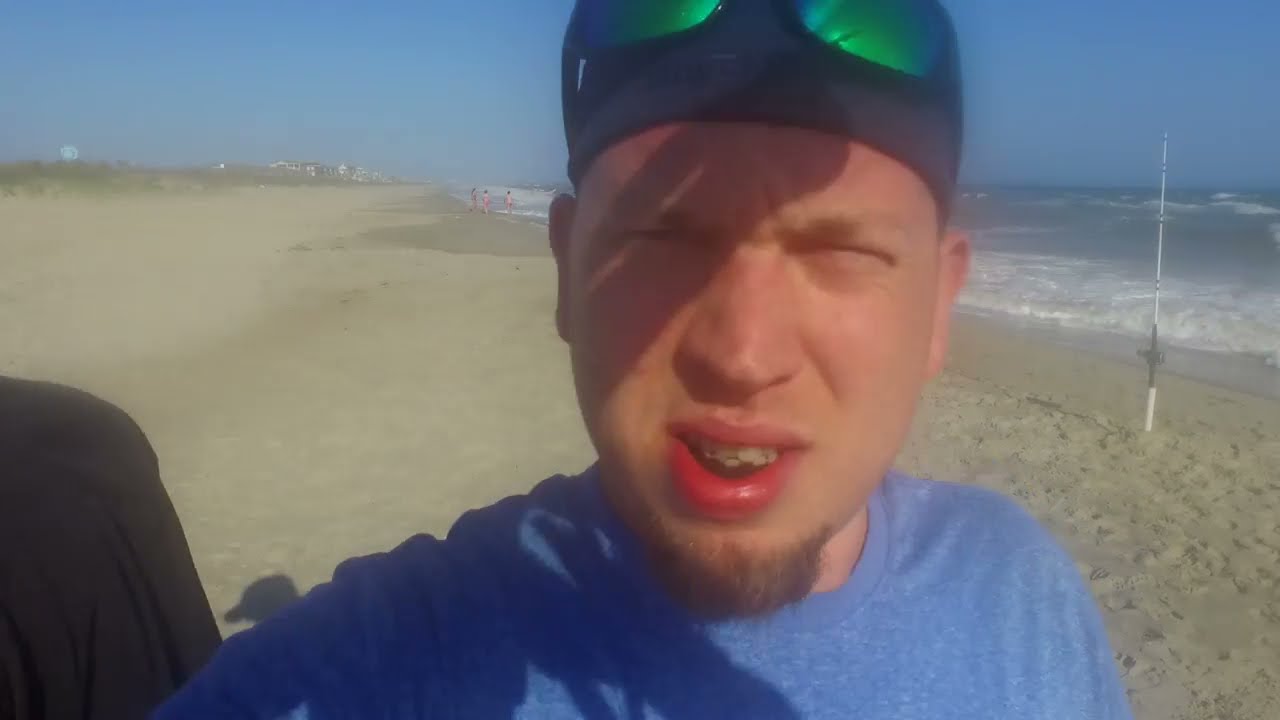A white man with a goatee takes a close-up selfie at the beach, framed by the sunlit, sandy shore and the blue ocean waves crashing in the background. He wears a blue t-shirt and a dark-colored hat backward, with green sunglasses perched on top of it. His expression shows squinting eyes, likely from the bright sunlight, and an open mouth revealing teeth that appear uneven and possibly braced. There are buildings visible in the far distance and people wading into the water, playing on the beach. To his right, a person in a black shirt is partially visible, along with a white and black fishing pole planted in the sand. The image, captured under a clear blue sky, is slightly blurry, and while rich in descriptive detail, it may not be the best for social media.